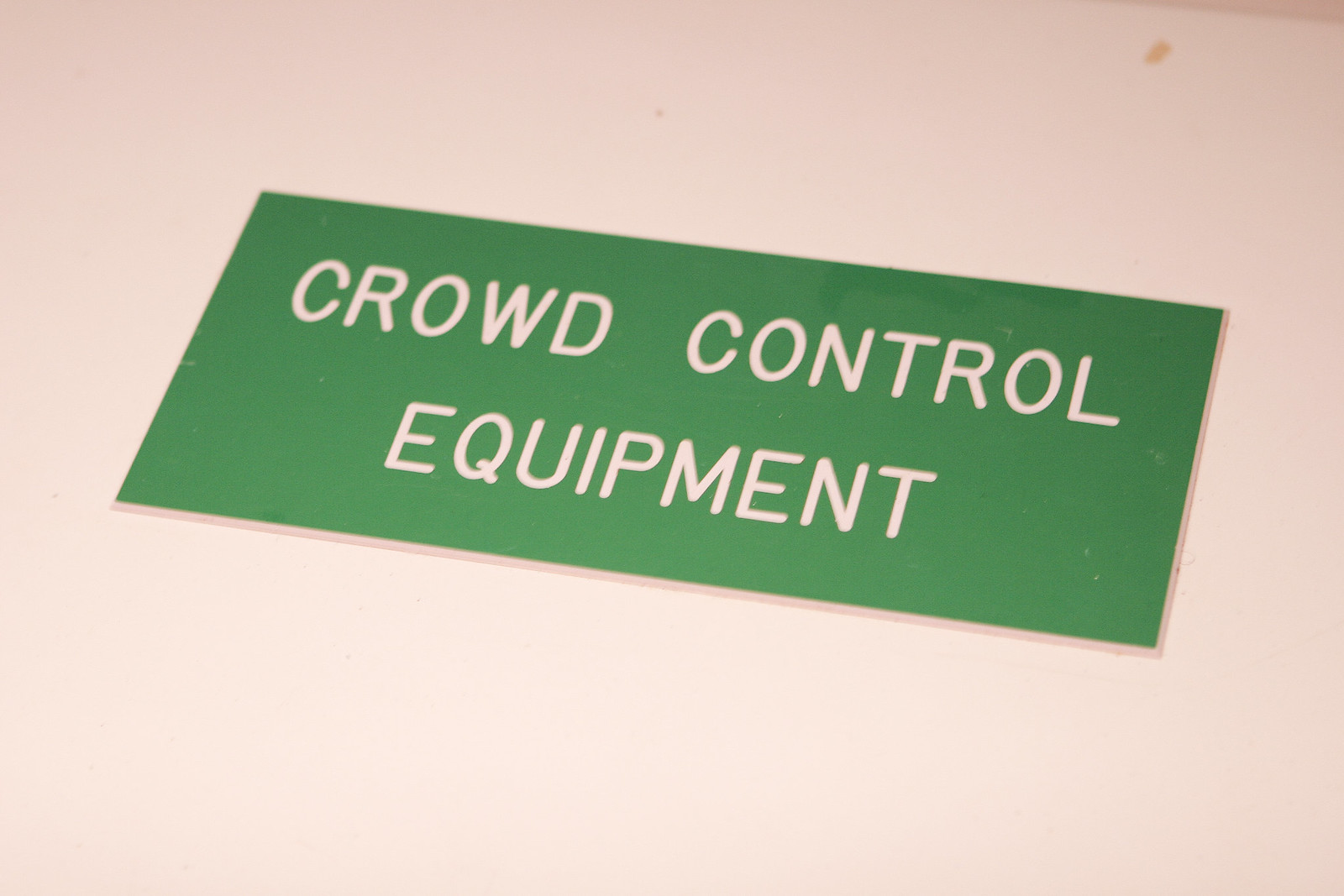The image depicts a medium green rectangular sign with white text that reads "crowd control equipment." The sign is slightly tilted so that the top left corner is elevated higher than the bottom right corner. It is situated on an off-white or light pink flat surface that is mostly plain, though there is a slight yellow stain near the top right corner. The font of the text is simple and rounded, resembling Arial. The sign and the surface it lies on are the main focus, with the surface appearing somewhat dingy in places.